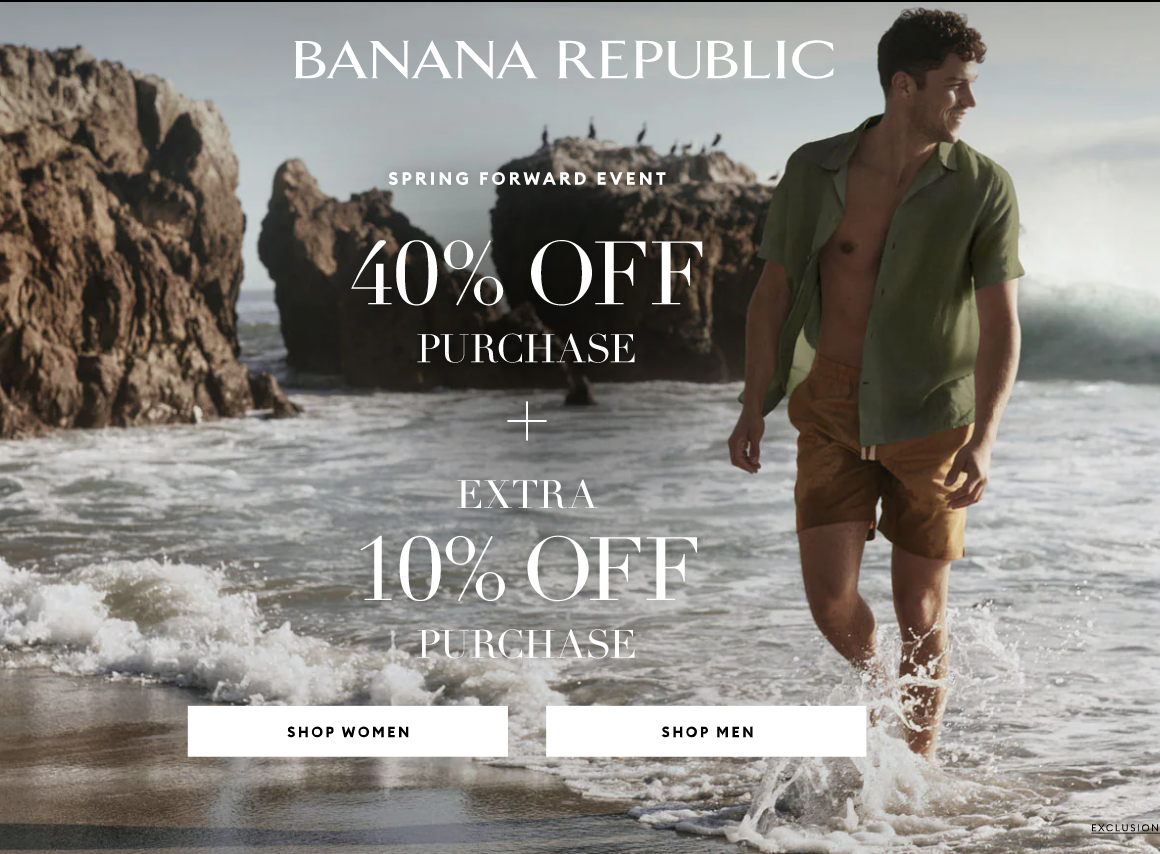The image depicts a scenic coastal landscape used as a backdrop for a Banana Republic advertisement. The scene is set outdoors under a slightly overcast sky, lending a grayish hue to the background. Below the sky lies a vast ocean, with rolling waves gently cresting against the shoreline. The wet sand traces the boundary between the water and the rugged terrain adorned with large, jagged rocks that stretch from the left edge of the image to a little past the center.

Prominently featured at the top center of the image are the words "Banana Republic" in bold, white capital letters. Beneath this, the text announces the "Spring Forward Event" and highlights promotions: "40% Off Purchase" and "Plus Extra 10% Off Purchase," all in bold print. Below these promotional texts, there are banners on white backgrounds with black text that read "Shop Women" and "Shop Men."

In the foreground, adding a personal touch to the advertisement, is a man walking through the water. He is dressed in shorts and an open, short-sleeve button-down shirt, looking over his left shoulder, which adds a sense of casual, relaxed elegance to the scene.